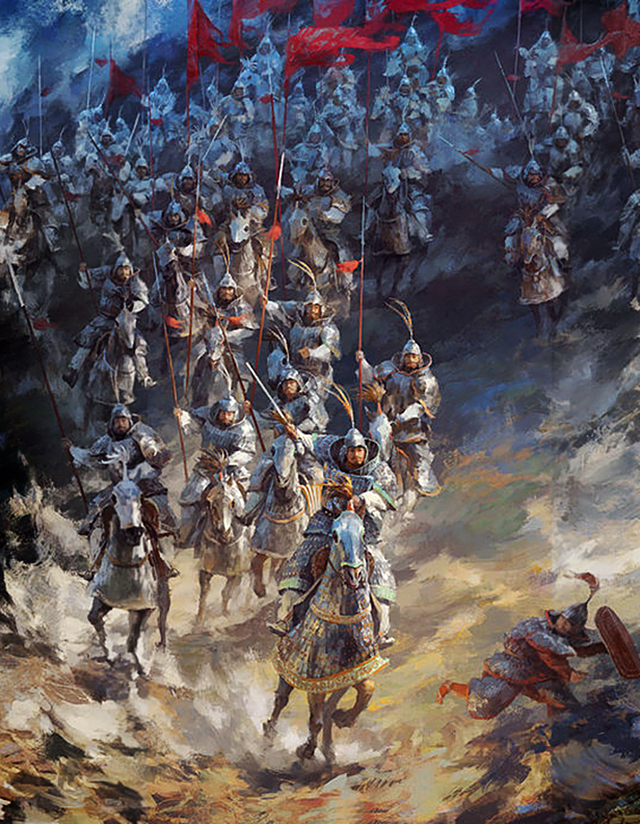This painting vividly captures the chaotic intensity of a historic battle scene. A throng of warriors on horseback, all clad in protective armor and medieval costumes complete with helmets, charges down a hill and into the foreground. The horses, draped in material that covers them down to their legs, emphasize the era's attention to both offensive and defensive measures in warfare. Each warrior brandishes a spear, and numerous red flags are held aloft, signaling the unity and ferocity of their advance. The scene contrasts light and dark: the upper part of the image is shadowed, perhaps by the incline, while the lower foreground is brightly illuminated, underscoring the dramatic descent into battle. Amidst the tumult, a figure is captured in a moment of desperation, diving and glancing back in fear as they try to escape the oncoming cavalry. Patches of blue and water elements add further depth and movement to this historical tableau, imbuing the painting with a sense of impending action and urgency.